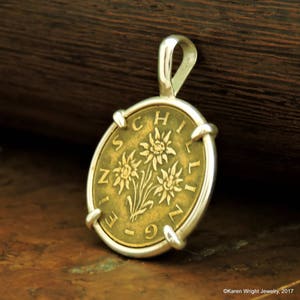The image depicts a detailed gold pendant likely designed for a necklace. The pendant is oval-shaped with an ornate hook at the top and lies diagonally against a dark brown background that features light gold striations. The solid surface beneath the pendant has small patches of light green, adding texture. Propped against what appears to be a dark, granite-like or wooden surface, the pendant displays the inscription "EINSCHILLING" encircling its outer edge. At the center of this gold oval, which has a subtle yellowish tint, three abstract flowers are intricately carved. In the bottom right corner of the image, a small text reads "January 2017," although the first two words are indecipherable.